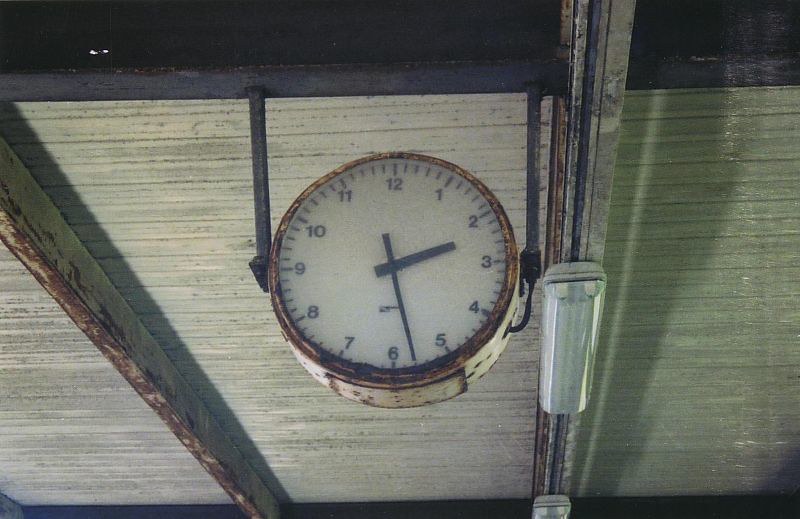This is a photograph of an old, rusted clock that appears to be situated in an aging building, possibly reminiscent of a train station. The clock, with a white face, displays the time as 2:28. It is suspended from the cream-colored, wooden plank ceiling by two metal rods, which also possibly house the electrical wiring for the clock. The ceiling supports are visible with exposed wooden rafters and beams. Some of the wood exhibits a greenish tint. On these beams, there are fluorescent tube downlights attached, which add to the sense of disrepair. The overall setting, with its metal sheet roof covering visible from below and the antiquated condition of the clock, suggests this is in a well-worn, utilitarian space.